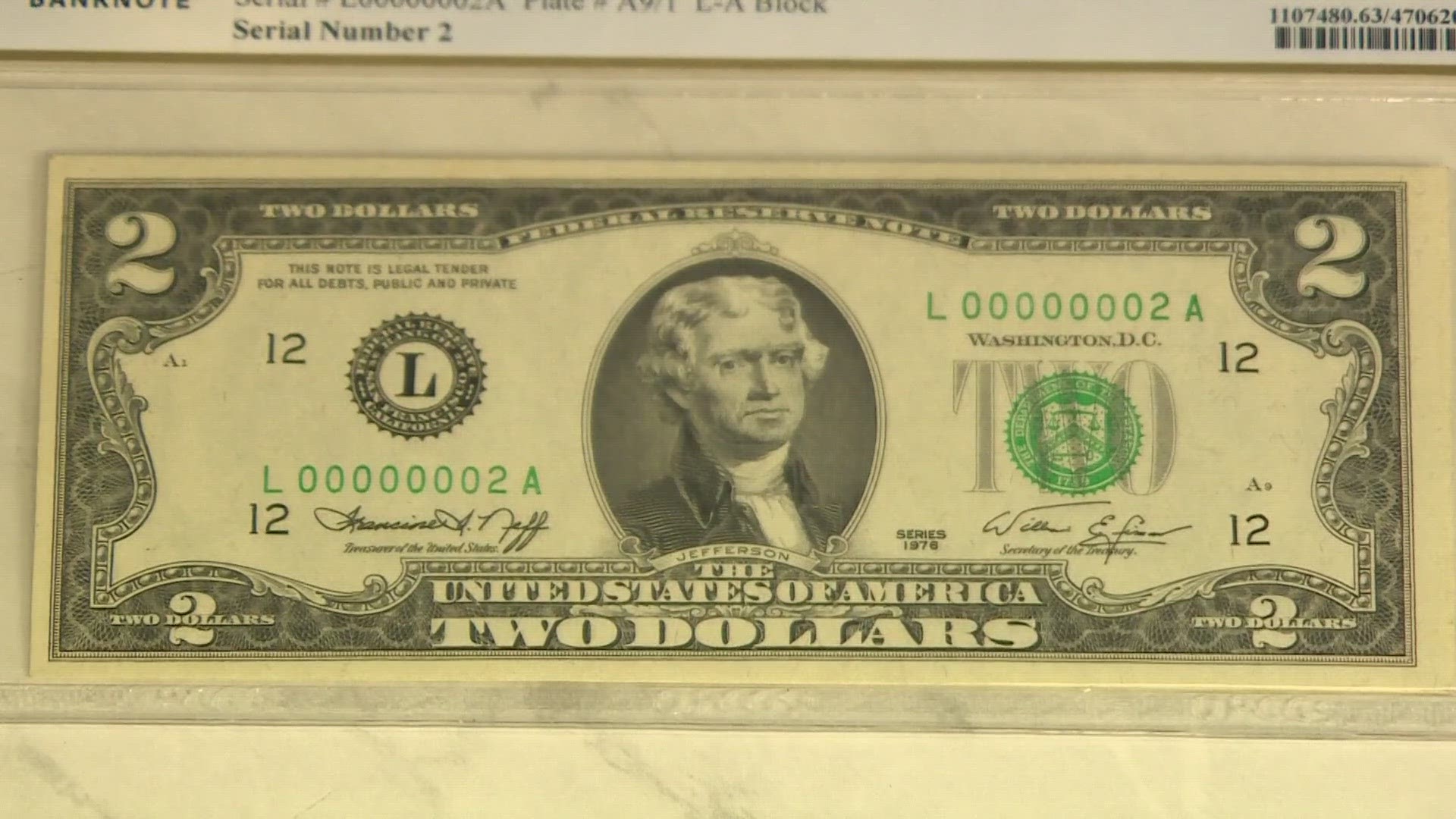This detailed image depicts a $2 bill, predominantly showcasing the face side of the currency, encased in a plastic frame. In the center of the bill is a portrait of Thomas Jefferson, clearly labeled "Jefferson" beneath his image. Each corner of the bill prominently displays the number "2" indicating its denomination. The bill is predominantly black, gray, and white with a slight greenish tinge. The top of the encasing sheet features printed text, including "serial number 2" and the word "banknote," along with a barcode located in the upper right corner. To the left side of the bill, there are green markings including an "L," followed by a series of zeros, a "2," and an "A." On the right side, there is an image of a seal with numbers displayed above it. The bill is framed, suggesting that it is being preserved or displayed, possibly highlighting its value or uniqueness.